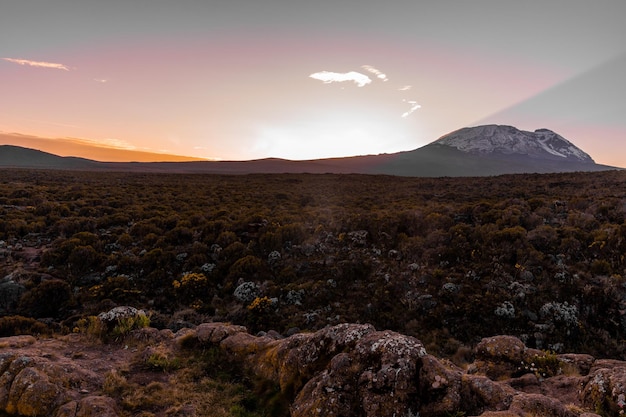The image depicts a serene outdoor landscape at either sunrise or sunset, showcasing a vast, arid field dotted with small bushes, grasses, and a few green trees. In the foreground, brown rock formations add texture to the scene. The backdrop features a distant mountain range and a prominent tall hill that transitions into a rocky mountain on the right. The sky exhibits a gradient of hues, from the grayish tones to vibrant pinks and oranges, with the sun partially visible over the mountain peaks. A few clouds scatter across the sky, enhancing the tranquil atmosphere of the scene.